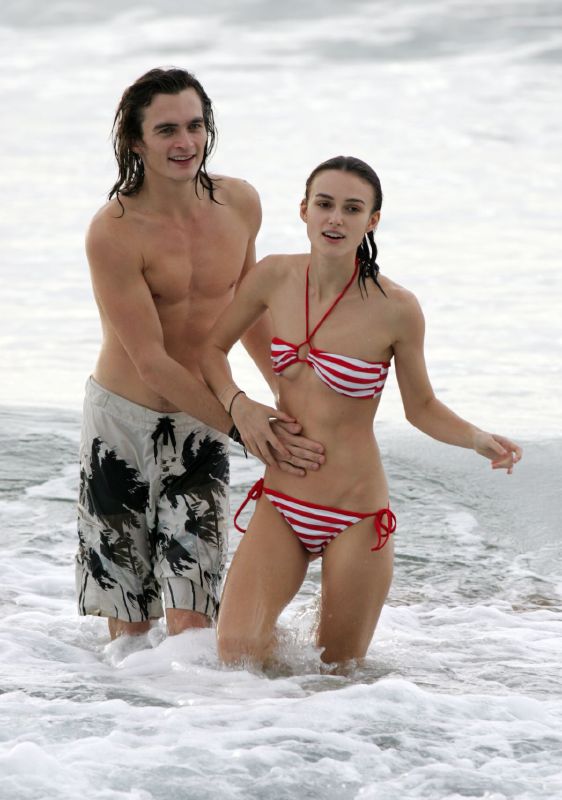In this photograph, a young couple is knee-deep in the ocean, surrounded entirely by water with no visible shoreline. The young man, with shoulder-length wet brown hair, is bare-chested and wearing white board shorts adorned with black palm tree patterns. The young woman, who bears a resemblance to Keira Knightley, has slightly past shoulder-length wet brown hair and is dressed in a red-and-white horizontal-striped bikini. The top of her bikini features a loop around her neck and narrow cups connected by a circle in the center, while the matching bottoms are tied at the hips. The man stands slightly behind her, his right hand gently placed on her stomach, over which the woman has laid her right hand. His left hand rests on her lower back, possibly offering support against the waves. Both are smiling softly, exuding a sense of closeness and enjoyment, perhaps on a beach vacation.